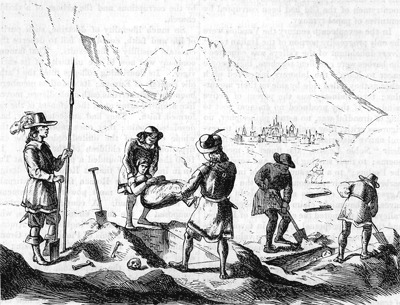The black and white drawing depicts a solemn burial scene set in what appears to be an era reminiscent of the 1500s or 1600s based on the style of clothing. The foreground features uneven ground scattered with bones and skulls. On the far left, a man stands guard, holding a long spear and gazing to the right; his attire includes a hat with a feather, evocative of old-time costumes possibly seen in Robin Hood narratives. To his right, two men are lowering a woman into a freshly dug grave, their actions suggesting a somber ritual. Further right, two more men are actively digging another grave as part of the burial preparations. In the background, simple outlines depict distant mountains and a small, indistinct town or settlement nestled at the mountain's base. The absence of a detailed border emphasizes the stark and haunting simplicity of this historic scene.